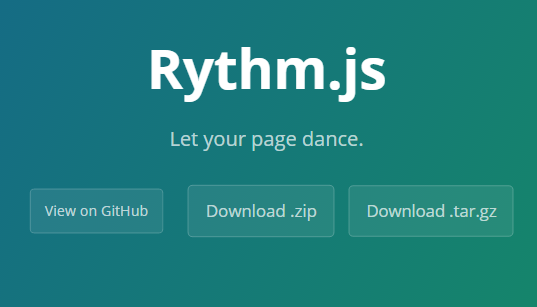This image is a screenshot of a webpage for a software program named "rhythm.js." The interface is artistically divided into two distinct color schemes: the left half features a dark green background, while the right half transitions into a brighter green with hints of teal and yellow. The header prominently displays the program's name, "rhythm.js," in large text at the top center of the page. Beneath this, a tagline in white text reads, "Let your page dance." Below the tagline are three horizontal, rectangular buttons arranged from left to right. The leftmost button is labeled "View on GitHub." The central button reads "Download the .zip file," and the far-right button is labeled "Download .tar.gz." This layout and design elements suggest a user-friendly interface aimed at providing easy access to resources and downloads for the rhythm.js program.